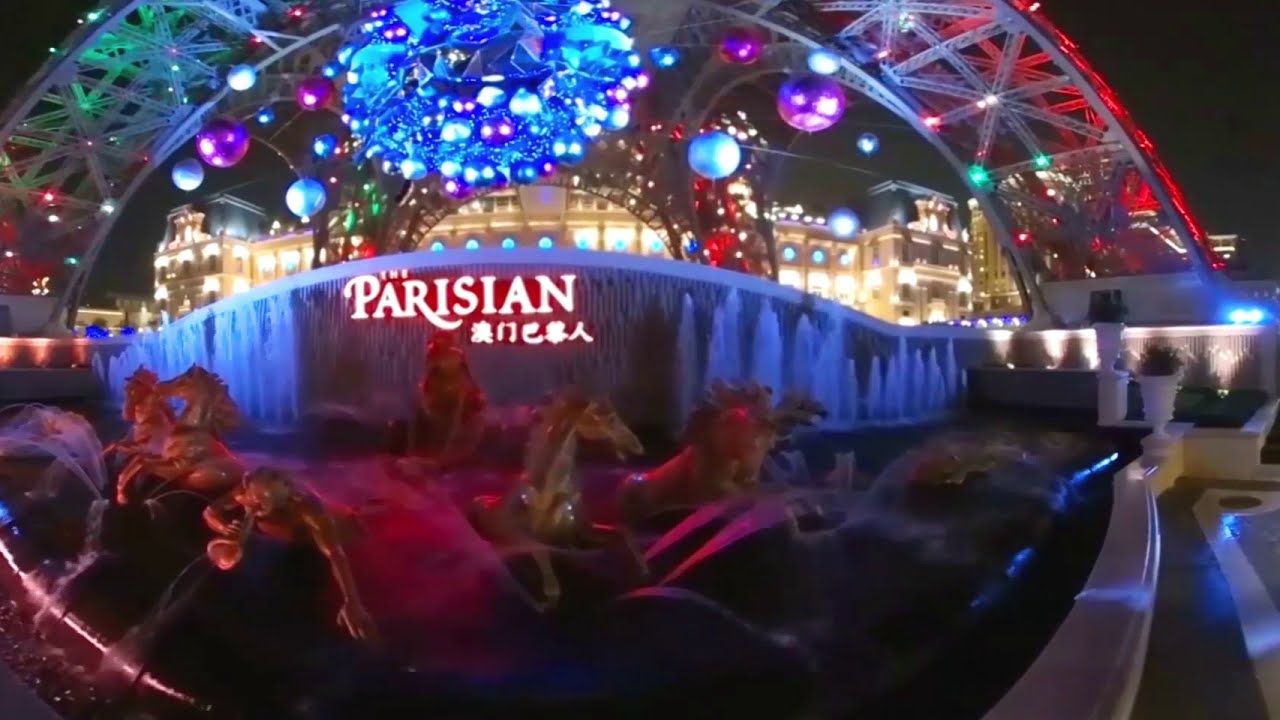Under the pitch-black night sky, a grand, ornate water fountain stands majestically in front of a well-lit, towering building, possibly a resort or palace. The centerpiece of the fountain features multiple golden-colored horses depicted in mid-gallop, with water dramatically pouring from beneath their hooves. A striking statue of a person blowing a horn rises among the horses, with water streaming elegantly from the horn. Vertical streams of water shoot up high from the fountain's back wall, complemented by cascading water from a higher tier. A prominent LED sign reading "The Parisian" illuminates the scene, accompanied by additional text in Asian script. Encasing the bottom of the fountain pool is a white barrier, while an ornate metal archway adorned with large purple and blue globes and intricate light displays arches over the scene, adding to the festive atmosphere. The entire setup, including lights and decorations, gives the impression of a grand event or festival, accentuated by the glistening water and vibrant lights.